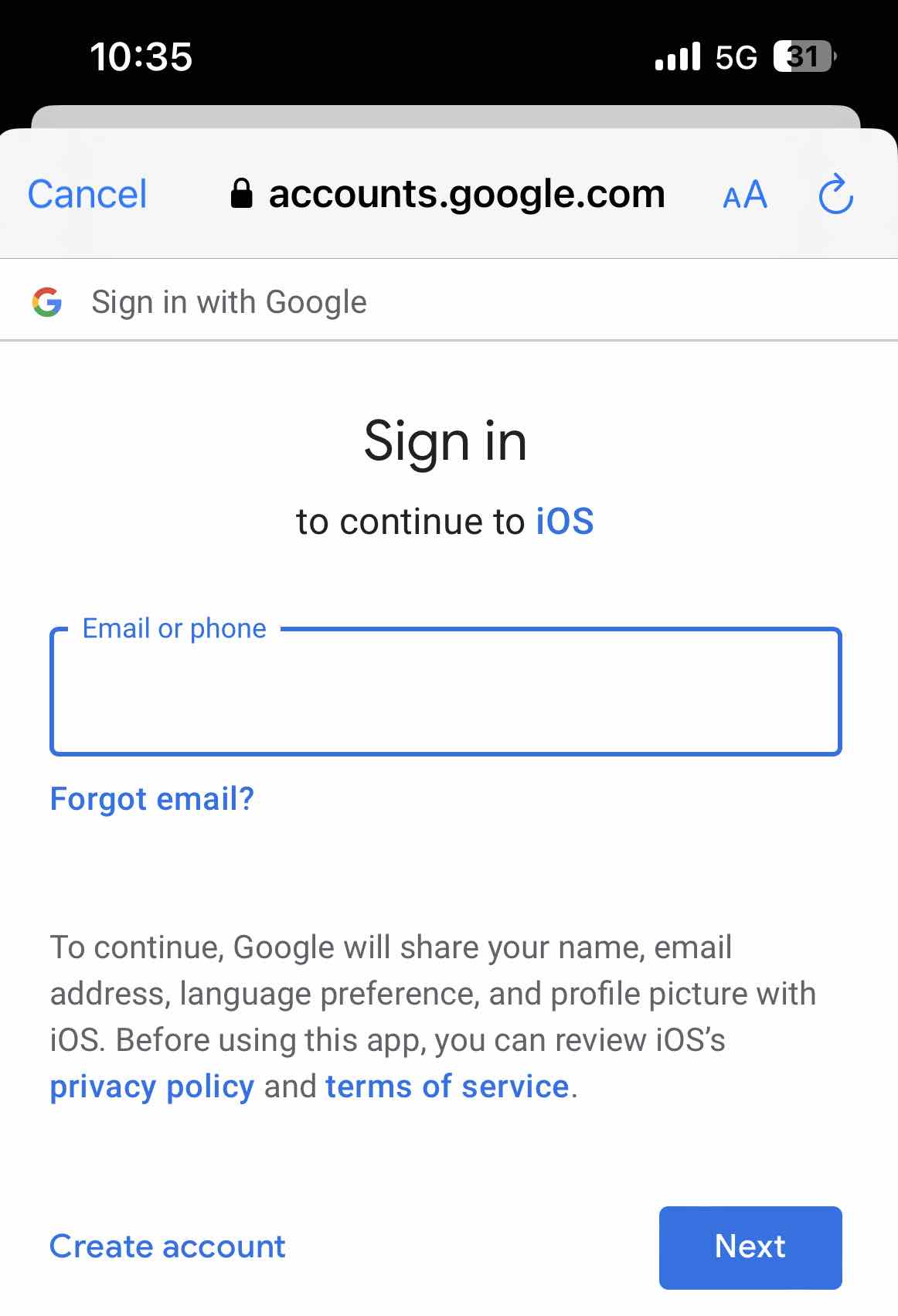This image is a screenshot captured in portrait mode. The background is predominantly white, with a black strip at the top. 

- **Top Row:**
  - **Left Corner:** Displays the time "10:35."
  - **Right Corner:** Indicates the battery level at "31%."

- **Second Row:**
  - The word "Cancel" appears as a clickable link in light blue on the left.

- **Third Row:**
  - **Center:** The URL "accounts.google.com" is shown.
  - **Right Side:** Features options such as font size controls in blue and a reload arrow.

- **Fourth Row:** 
  - Following the Google logo, there is a sign-in instruction: "Sign in with Google."

- **Main Section:**
  - **Header:** In large black letters, "Sign in" followed by "to continue to iOS" with "iOS" in blue.
  - **Input Field:** A blue outlined form field labeled "Email or phone" where users are expected to fill in their credentials.
  - **Forgot Email Link:** A clickable blue link labeled "Forgot email?"

- **Information Section:**
  - "To continue, Google will share your name, email address, language preferences, and profile picture with iOS. Before using this app, you can review iOS's privacy policy and terms of service," both phrases appear as clickable blue links.

- **Bottom Row:**
  - **Left Corner:** A blue link labeled "Create account."
  - **Right Corner:** A light blue button labeled "Next."

Overall, this screenshot depicts an iOS device prompting the user to sign into their Google account with options to create an account or proceed by clicking the "Next" button. The interface elements are interactive, providing a seamless and intuitive user experience akin to real-life interaction.